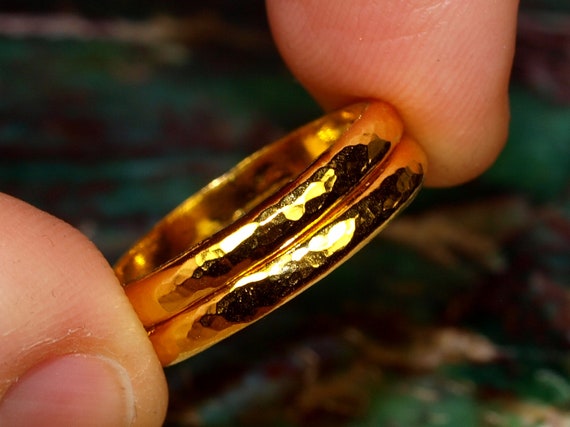This detailed, close-up color photograph captures the interplay of light on a pair of intertwined gold rings. Positioned between an index finger and thumb, the rings exhibit a hand-hammered texture with rough, faceted surfaces that lend them a rustic charm. The gold bands, almost identical in size and stacked atop one another, radiate a warm, 18-karat golden glow. The fingers, pale in complexion, hold the rings with the thumb at the bottom left and the index finger behind, creating a diagonal orientation from the upper left to the bottom right. The background is blurred, featuring a greenish-brown, mottled texture, possibly a tablecloth, enhancing the focus on the glittering, reflective rings. The fingers and the rings are the sole subjects, with no other persons or animals present.